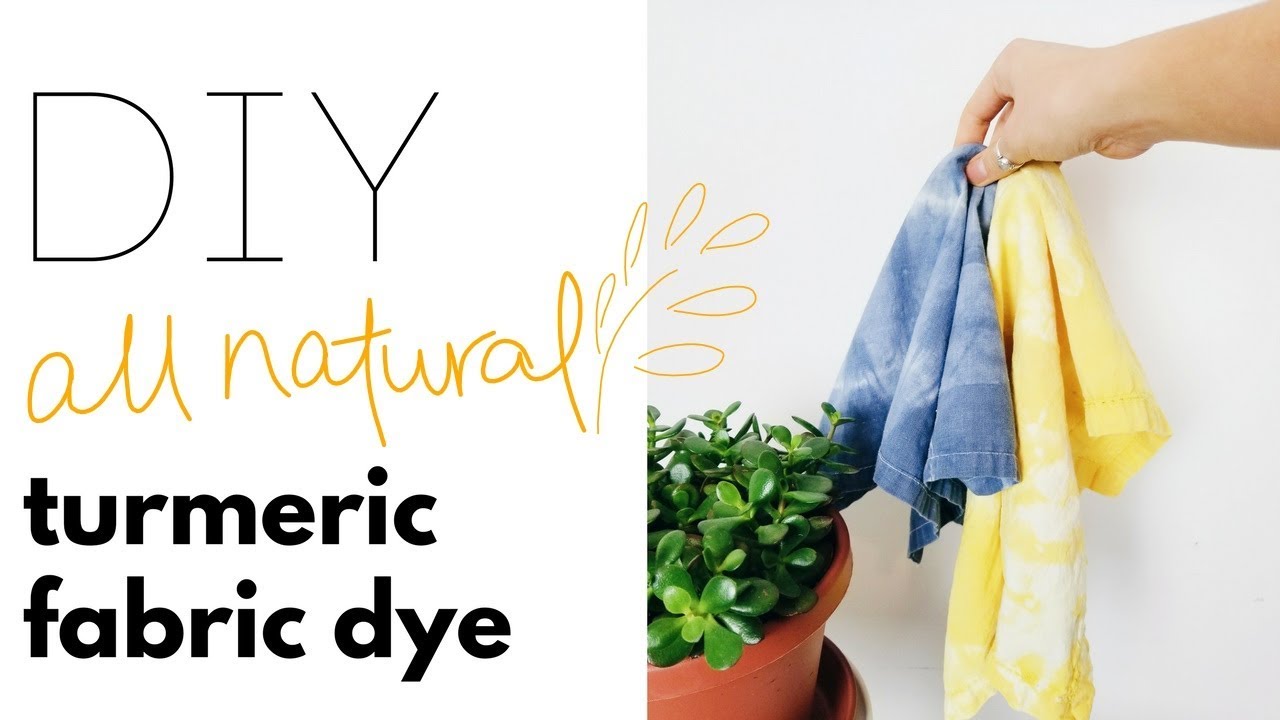The image is divided into two sections: a textual part on the left and a photograph on the right. On the left side, the word "DIY" is prominently displayed in thin uppercase letters, followed by "all natural" in gold cursive lowercase letters, accompanied by an illustration of a single-stemmed, six-petal orange flower to the right of the letter "L." Below this, "turmeric fabric dye" is written in bold black lowercase letters, with "turmeric" stacked above "fabric dye."

The right side of the image showcases a photograph featuring a white hand and part of the forearm holding two pieces of clothing against a white background. The left piece of clothing is a smaller blue towel, and the right one is a larger yellow towel. The hand, adorned with a thumb ring, is positioned near a potted green succulent plant, which looks almost plasticky. The plant is housed in a round, orange pot. The setting exudes a DIY vibe, underscoring the natural approach to fabric dyeing using turmeric, likely for the yellow towel.